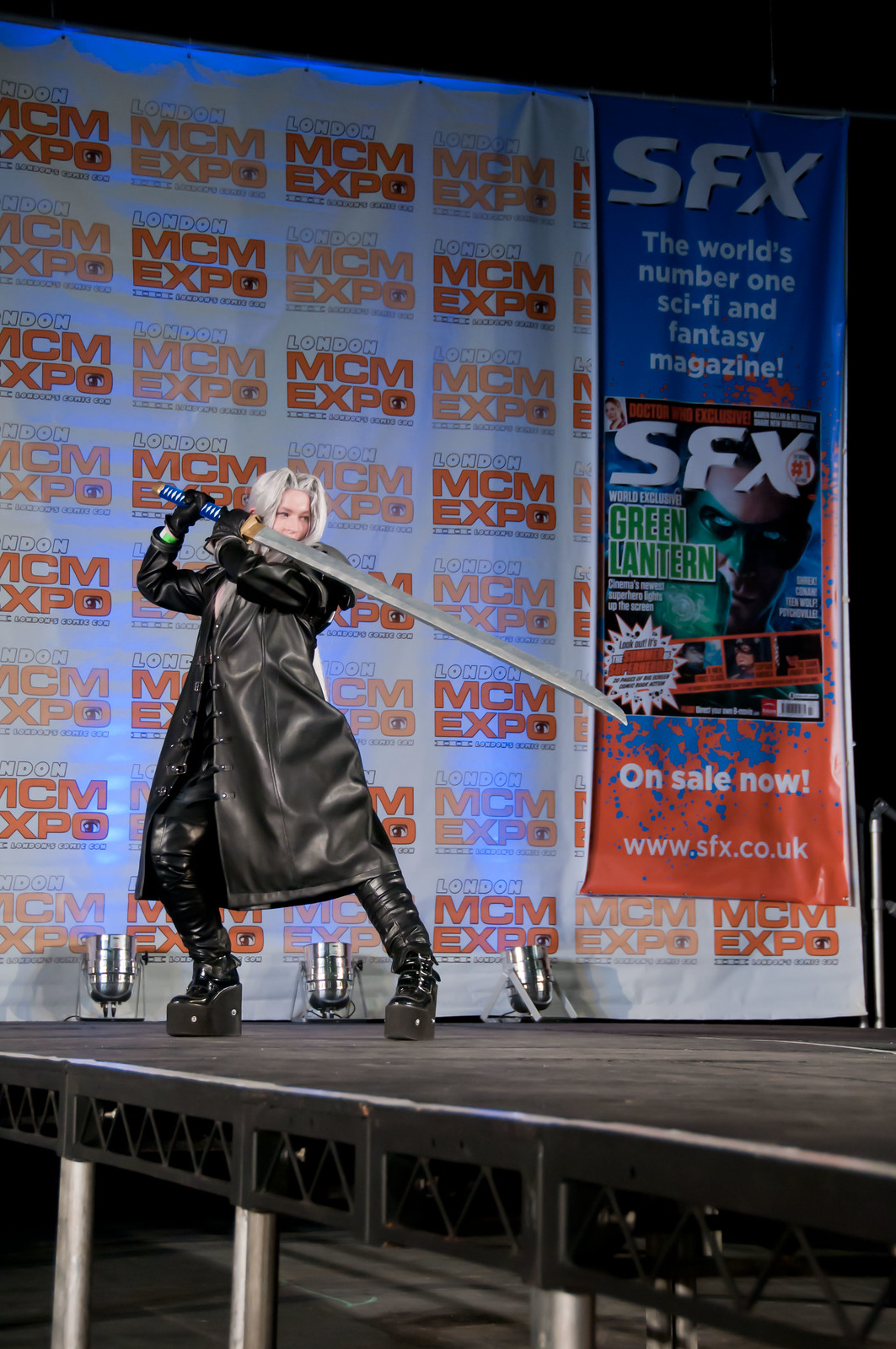This detailed photo captures a moment at what appears to be an anime or comic book expo. The scene is set on a stage illuminated by spotlights, where a person stands dressed as Sephiroth from Final Fantasy VII. The character’s iconic look is meticulously recreated with tall platform boots, black leather pants, a long black trench coat, and a striking white wig. They hold an impressively long sword in front of them, adding to the dramatic effect.

Prominently visible in the background is a large white banner repeatedly displaying the text "London MCM Expo" in a combination of white and orange. Another banner on the far right, predominantly blue and orange, advertises SFX, described as the world's number one sci-fi and fantasy magazine. This banner includes an image of the magazine and additional text reading "On Sale Now" followed by the website www.sfx.co.uk. The stage itself is noticeably elevated, situating the cosplayer well above the event floor, enhancing the overall grandeur of the presentation.